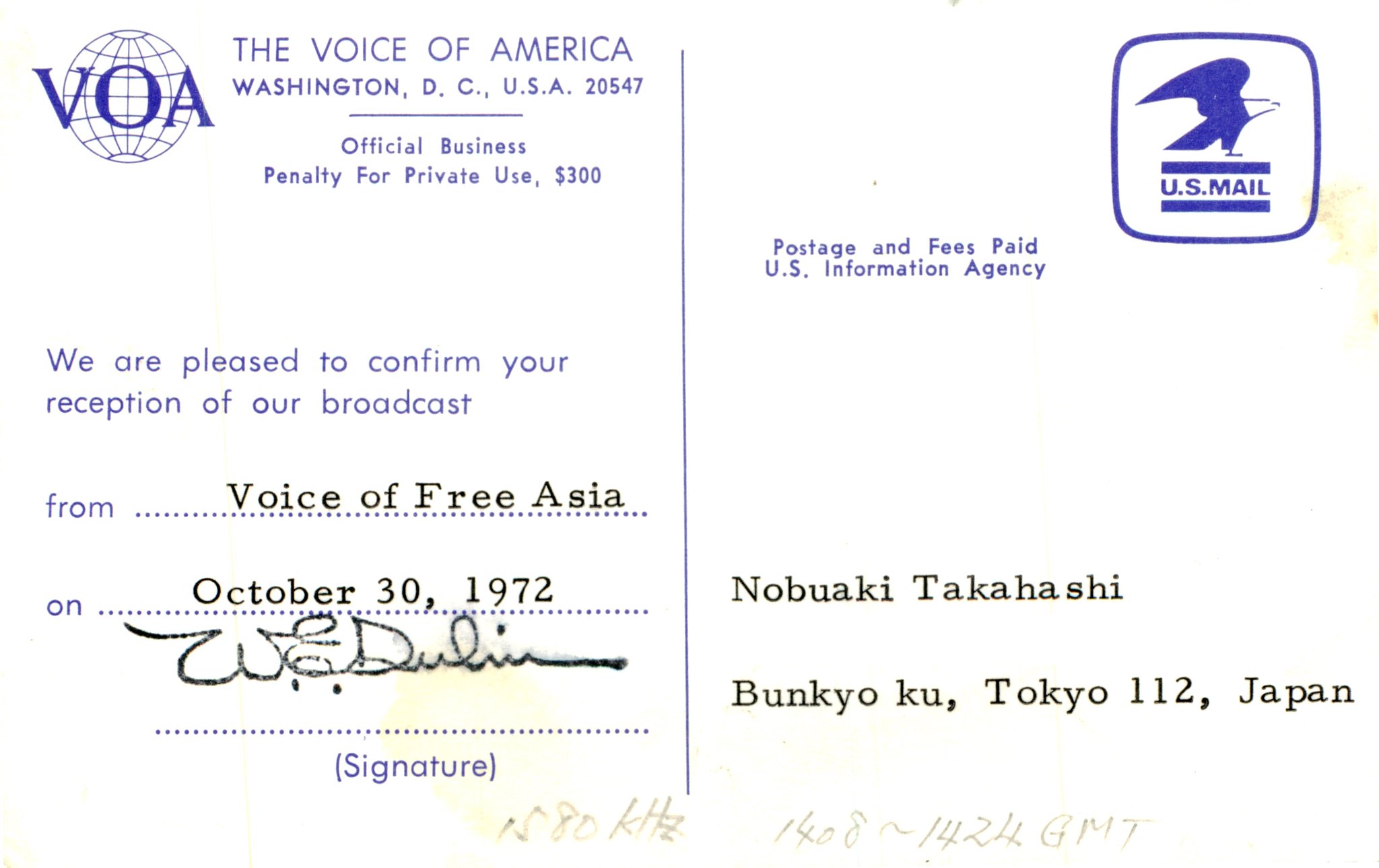The image depicts a vintage postcard, likely a photocopy, characterized by distinct elements and text in both blue-purple and black fonts. At the top left corner, the logo of "The Voice of America" includes a circular earth symbol intersected by horizontal and vertical lines accompanied by the letters "V-O-A." Below this, the postcard reads: "The Voice of America, Washington, D.C., USA, 20547, Official Business, Penalty for Private Use, $300." In the center left, a confirmation message states: "We are pleased to confirm your reception of our broadcast from Voice of Free Asia on October 30, 1972," followed by a cursive signature, "W.E. Doolin," noted as a signature in parentheses. On the right side, the vintage U.S. Mail logo featuring a perched eagle is present, with text that reads: "Postage and Fees Paid, U.S. Information Agency." Below this, in black text, it lists the recipient's name and address: "Nobuaki Takahashi, Bonkyoku, Tokyo 112, Japan." The white background of the postcard shows some yellowish stains, particularly noticeable at the top right and bottom center, and there is faint, mostly faded handwritten text at the bottom center of the image.